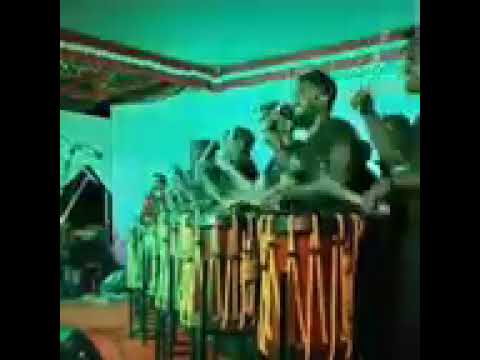The image, heavily obscured on the left and right sides by black vertical bars, features a very blurry scene that appears to be from a drumming concert. The central focus is a line of individuals, estimated to be between six and nine, possibly African or African-American men, who are playing tall, stand-up drums. These drums are predominantly brownish-orange with gradients that fade into yellowish-green hues. The entire photo is cast in a blue tint, which affects the colors of the background and the ceiling, the latter of which bears reddish decorations. The room itself is light-colored but appears bluish due to the lighting. Despite the blur, it seems that many of the drummers have their arms raised, indicating active drumming, and the backdrop is a light or white background that also adopts the bluish tone from the cast.